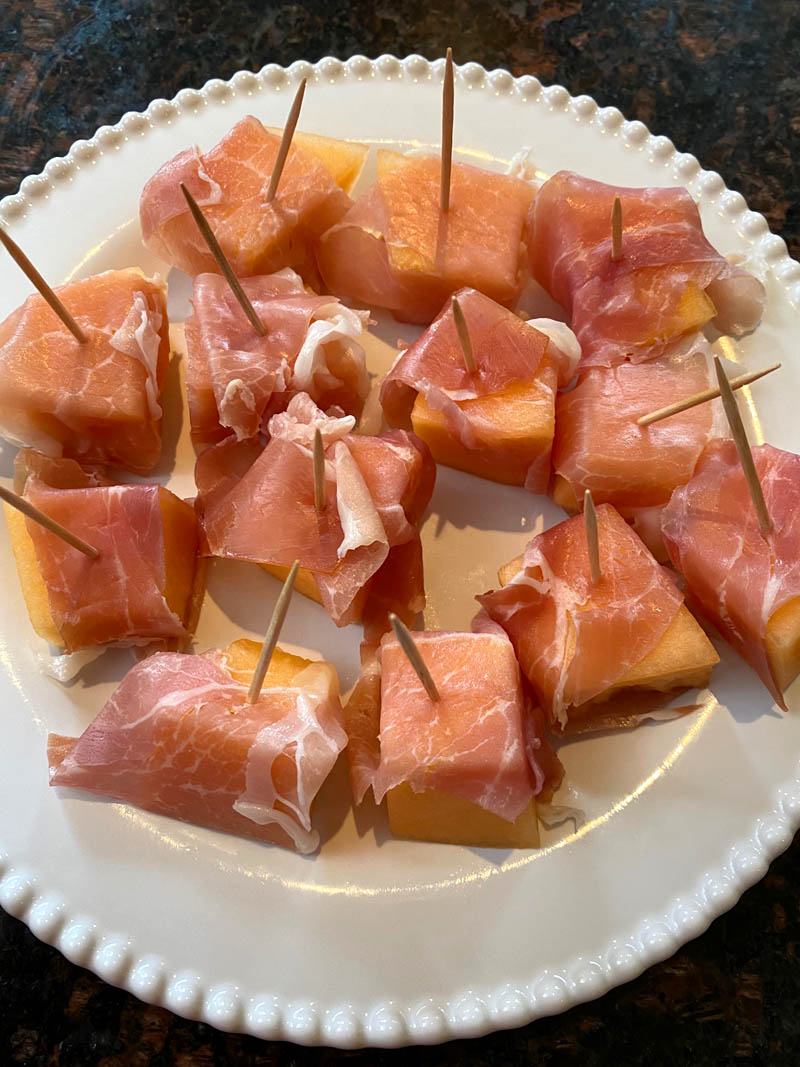This image features a close-up of a white, large, decorative plate with a beaded detail along its edge, arranged on a dark, possibly granite surface. The plate is predominantly filled with 13 appetizers, each consisting of yellowish-orange cantaloupe cubes wrapped in prosciutto or possibly salami, punctuated by protruding toothpicks. The toothpicks are arranged irregularly and skewer each prosciutto-wrapped cantaloupe, making them easy to handle as party snacks. Overall, the composition and presentation suggest these appetizers are intended for a social gathering.